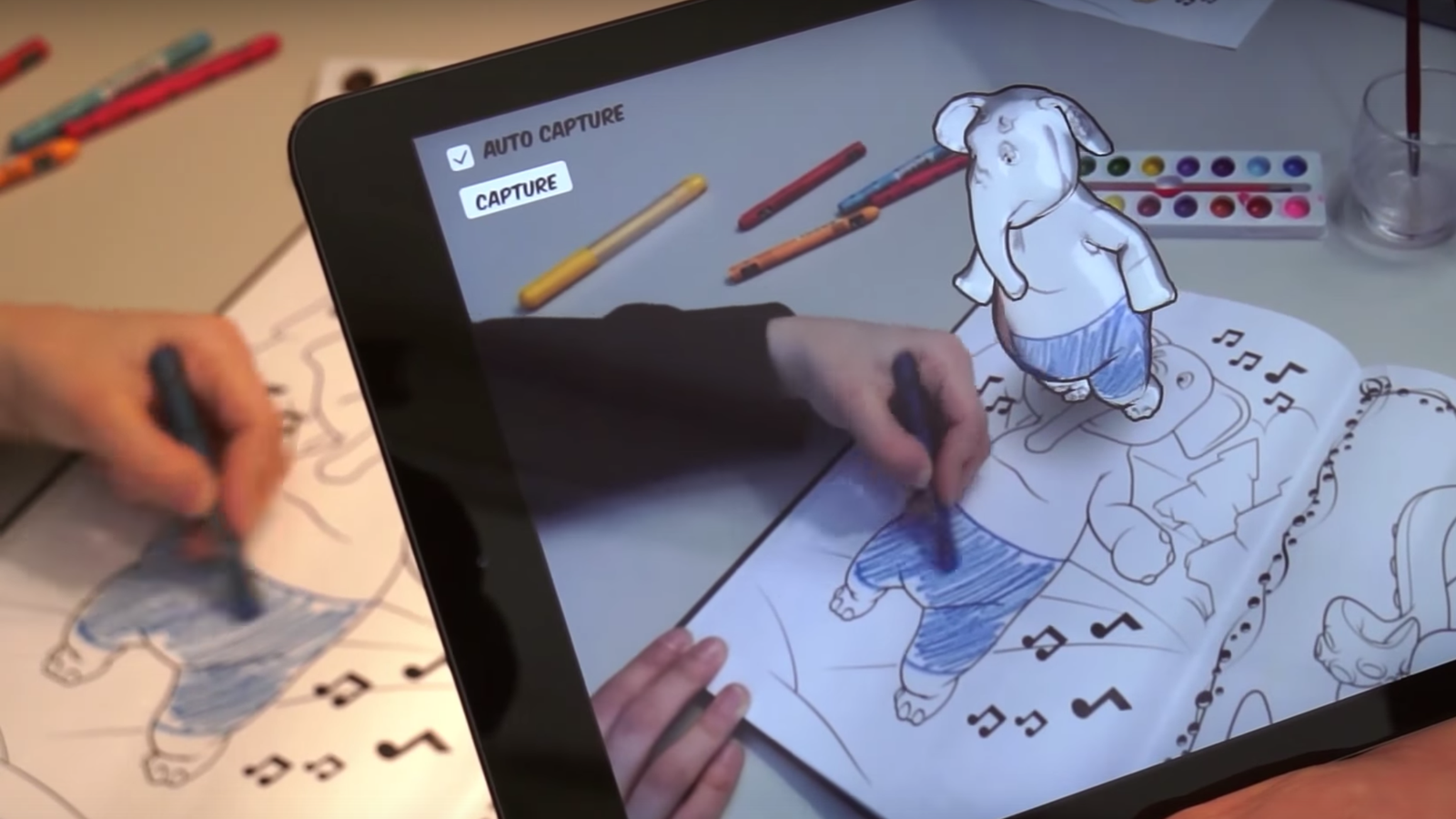The photograph captures a dynamic scene involving both traditional and digital elements of art. On the left side, a person with a blue crayon in their left hand, wearing a long-sleeved black shirt, is actively coloring an illustration of an elephant in a coloring book. The illustration includes the elephant wearing blue pants and surrounded by musical notes. Nearby on the white table are various art supplies, including crayons, paintbrushes, small paints, and a cup of water with a brush in it. 

On the right side of the photograph is a tablet screen displaying the same scene from a different angle. The screen shows the person's hand and the elephant illustration being colored. Additionally, the tablet screen presents a 3D render of the cartoon elephant standing on the coloring book page, mimicking the newly colored-in blue pants and sketchy coloring of the original drawing. In the top left corner of the tablet screen, "auto capture" is highlighted, indicating an automated photo feature, with a “capture” button situated below it. The use of digital enhancement brings the cartoon elephant to life, seamlessly blending traditional hand-drawn art with modern augmented reality.